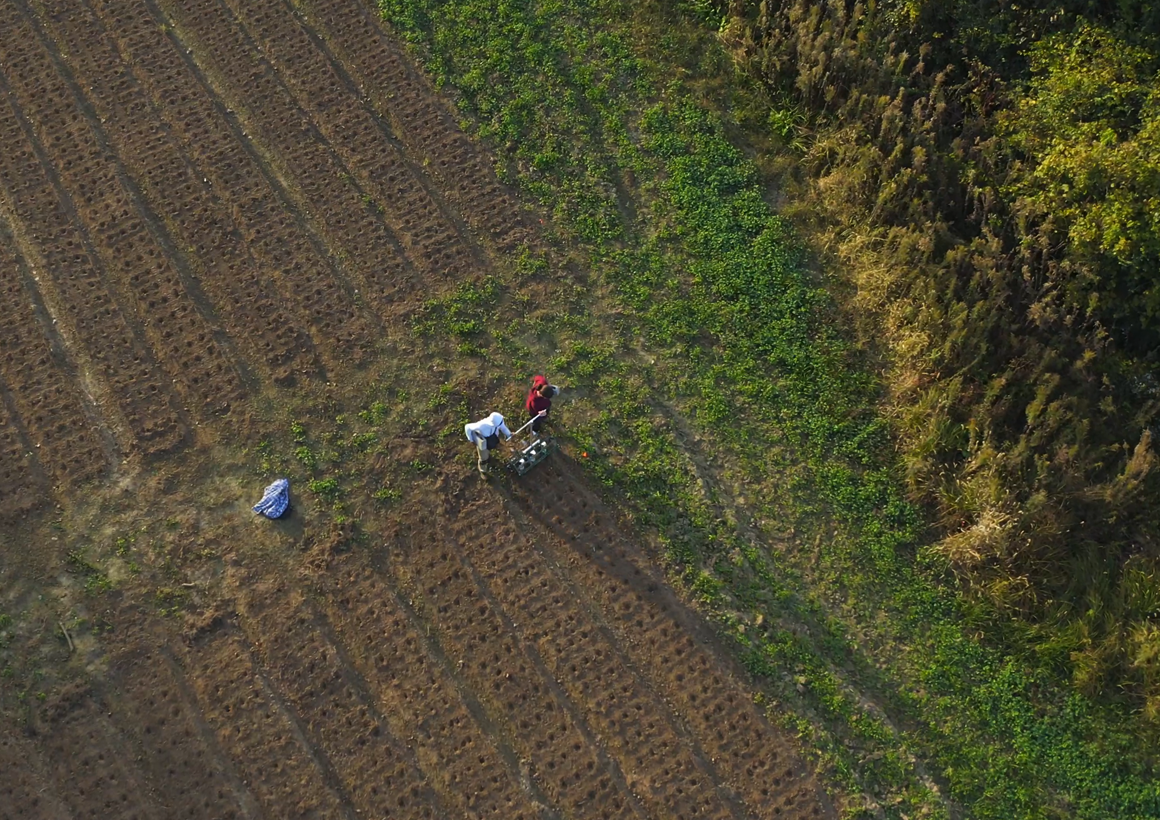An aerial photograph captures a farm field from above, revealing a richly detailed landscape below. In the upper right corner, a variety of green trees and short grass provide a lush backdrop. Spanning diagonally across the image from the center to the upper and lower left-hand sides, at least eight or nine meticulously plowed rows of dirt suggest that planting is underway, marked by equally spaced holes. At the center of this scene, three individuals stand out: one in a red shirt, another in a white shirt, and the third in a blue shirt. The figures in red and white are engaged in operating a metal contraption, likely a seeding machine, while walking along one of the dirt rows. To their left, the person in blue stands by, possibly supervising the operation. A blue object, potentially a bag or fabric, lies on the ground near them. The scene hints at the initial stages of agricultural activity, with both the human and natural elements captured in striking detail.